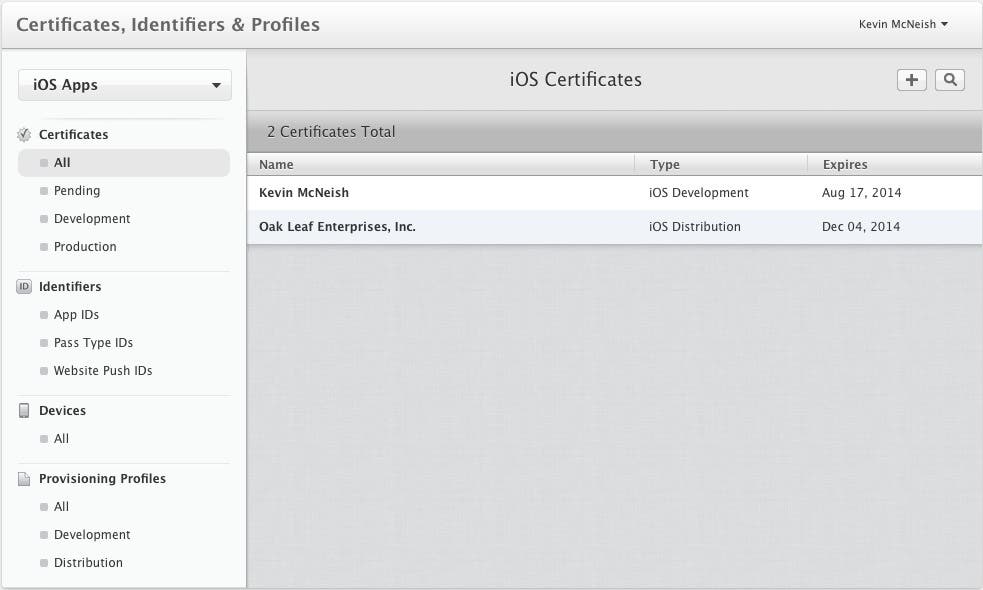The screenshot displays the "Certificates, Identifiers, and Profiles" section from a Mac operating system, specifically showcasing iOS certificates associated with Kevin McNeish (spelled M-C-N-E-I-S-H). At the top right, there's a drop-down menu with Kevin McNeish's name. The left side panel features a menu with tabs labeled "iOS Apps," "Certificates," "Identifiers," "Devices," and "Provisioning Profiles," each with various subsections like "App IDs," "Pass Type IDs," "Website Push IDs," "All Development," and "Distribution." The main section, titled "iOS Certificates," details two certificates: one indicates Kevin McNeish as an iOS Developer that expires on August 17, 2014, and the second belongs to Oakleaf Enterprises Inc. for iOS Distribution, expiring on December 4, 2014. The interface predominantly uses shades of white and gray, with a user-friendly layout that includes various checkboxes for sorting options.